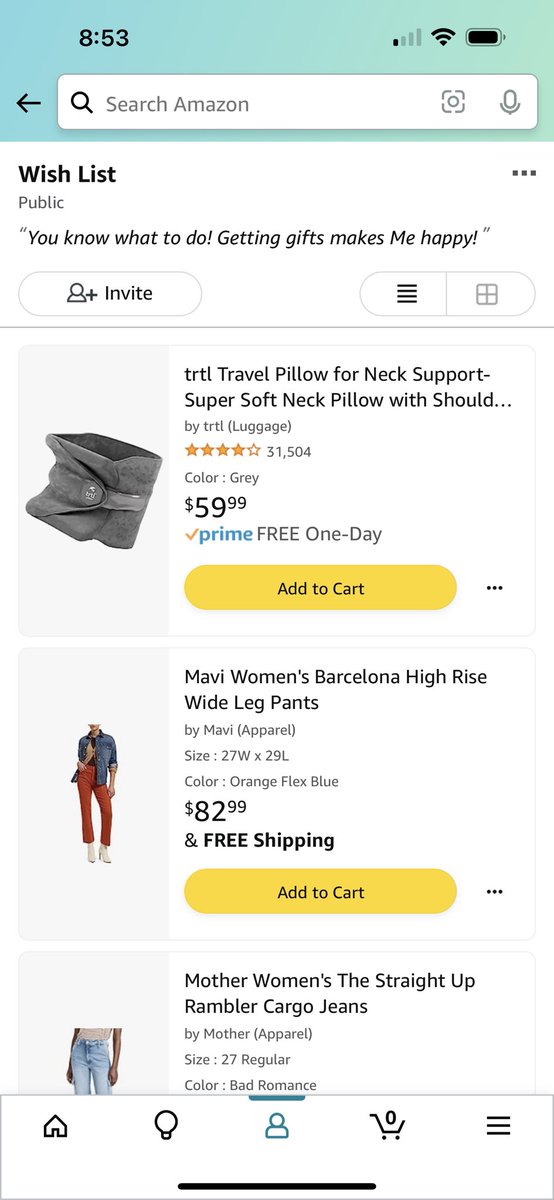In the image, we see a smartphone displaying an Amazon search page. At the top of the screen, there's a blue bar with the time displayed as 8:53 and a small black arrow pointing to the left. Below the blue bar is the search box, labeled "Search Amazon," and it includes icons for a camera and a microphone on the right side. The background of the page is white, and the text is predominantly black.

Beneath the search box, there's a section labeled "Wish List," which features three vertical dots on the right side. The list is marked as public with the statement, "Getting gifts makes me happy." There are two buttons below: one for inviting others, and another with a grid icon representing four quadrants.

The first product listed is a gray Turtle Travel Pillow for neck support, advertised as super soft and presented within a blue box. This item is priced at $59.99 and features a yellow "Add to Cart" button.

Following the travel pillow is a woman modeling Barcelona High-Rise Wide Leg Pants in a red color. These pants are priced at $82.99, with the detail of free shipping included. This product also has a yellow "Add to Cart" button.

The next item displayed is a pair of light-colored Mother Women's Straight Up Rambler Cargo Jeans.

At the bottom of the screen, there is a white navigation bar featuring icons for a home button, a search circle, a highlighted blue person icon, a shopping cart, and a menu represented by three horizontal lines. A black line underscores this navigation bar.